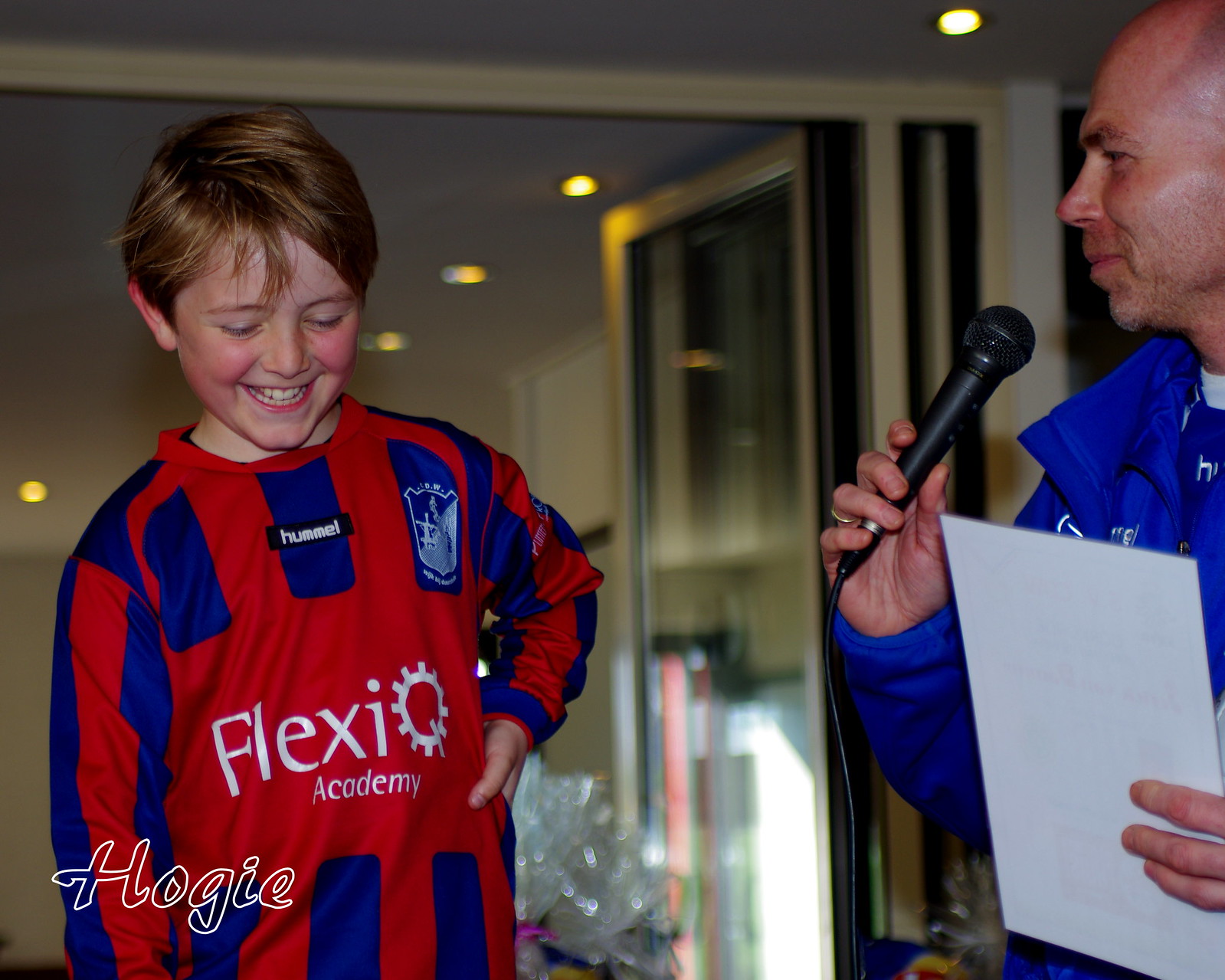The image captures a vibrant moment between a man and a child in an indoor setting illuminated by several small yellow spotlights on an off-white ceiling. The left side of the image prominently features a young boy with reddish hair, rosy cheeks, and a joyful laugh, looking downward. He is wearing a bright red, long-sleeved football jersey with deep blue stripes and white lettering that reads "FlexiQ Academy" at the center, alongside a white gear symbol. 

To the right of the boy stands a bald man with light skin and light whiskers, dressed in a bright blue sweatshirt. He holds a black wired microphone in his right hand and a script in his left hand, with a gold wedding band visible on his right hand. The man is looking towards the boy, appearing engaged in the moment. In the background, an open silver glass door bordered in silver is visible, along with some cellophane that hints at a gift. Adding a touch of personality to the image, the bottom left corner bears the word "Hoagie" in cursive.